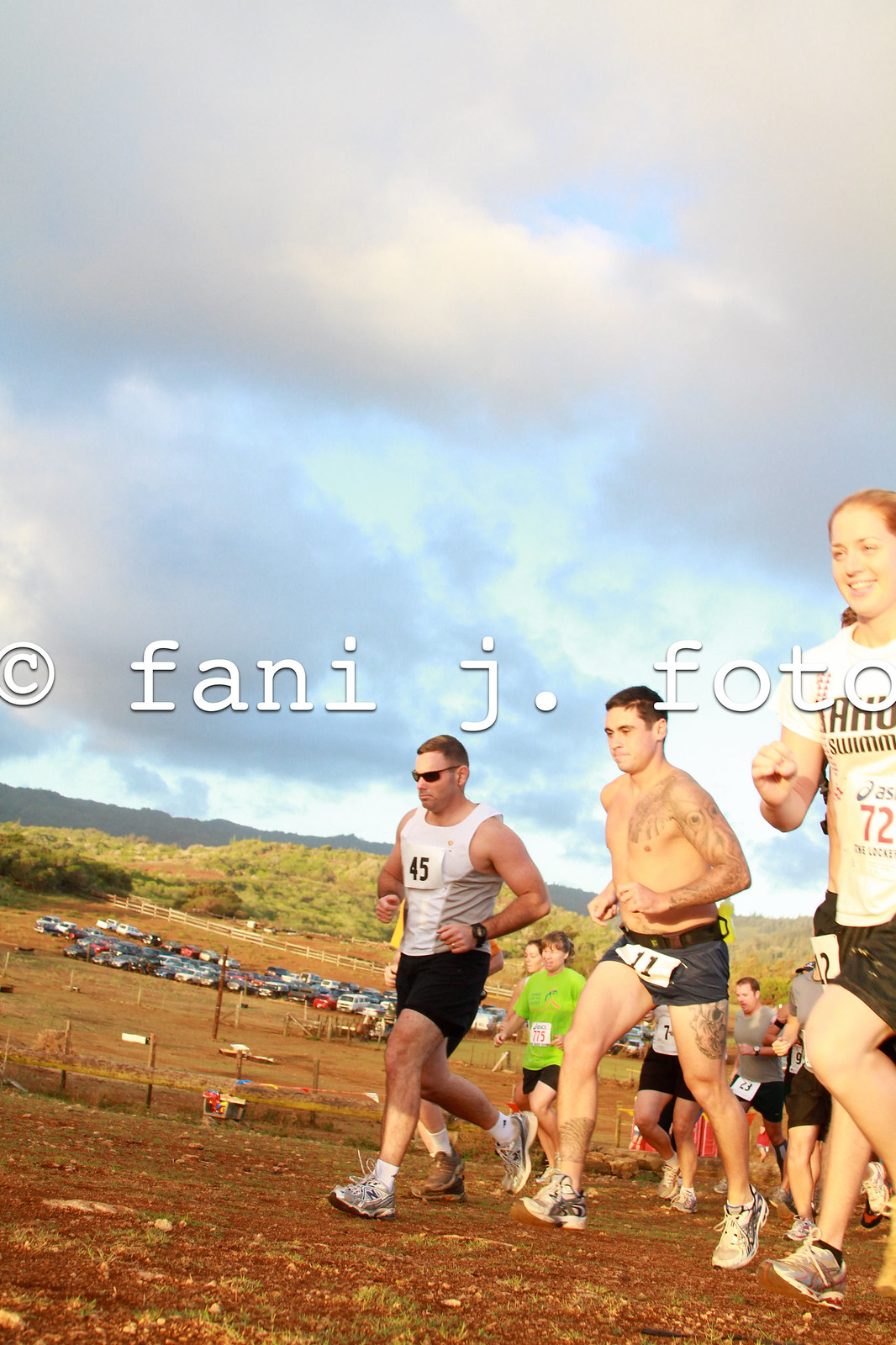In this photo, a group of about ten runners and walkers participate in what appears to be a marathon or charity race. The diverse group, which includes men and women, is running uphill on a slope comprised of reddish dirt with patches of grass. The sky above is mostly cloudy, with hints of blue peeking through, suggesting an overcast day with the possibility of rain. A distant hill and some trees add depth to the background, which also features a parking area with approximately 50 to 100 cars. Each runner is outfitted in black shorts and sporting numbers on their shirts or shorts: for example, one man wears a white tank top and black shorts with the number 45, another man has the number 11, and a woman is seen wearing a white shirt with black shorts and the number 72. A few runners are shirtless, and some display tattoos as they run with their hands to the sides. Across the middle of the image, large white text reads, "copyright Fannie J. Foto," adding an official watermark to the scene.